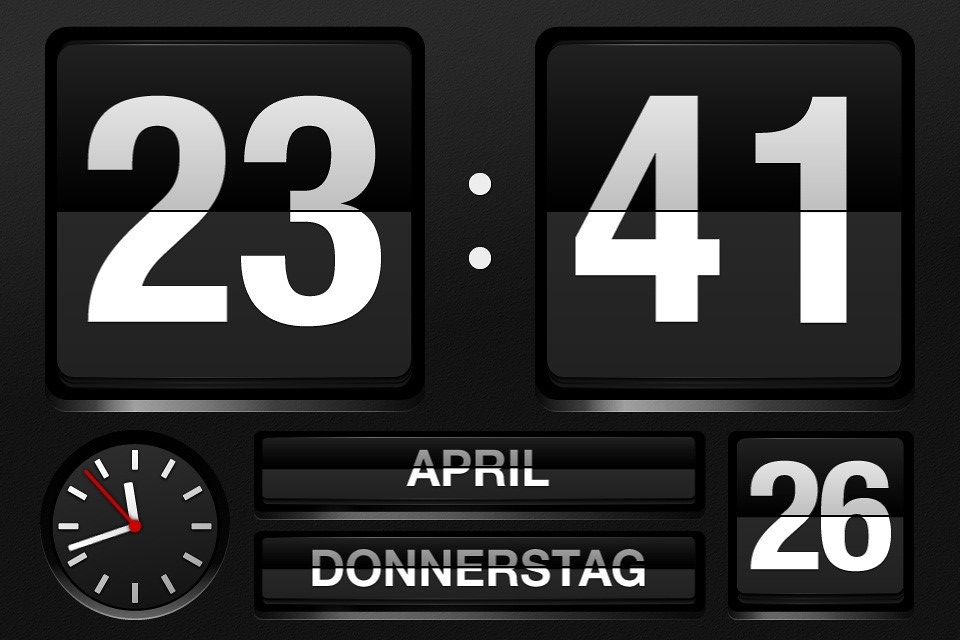This black-and-white photograph features a sleek, possibly AI-generated, digital-analog calendar clock. The entire device is a matte black, filling the frame. On the top left and right, there are black flip squares displaying "23" and "41" in large white font, separated by a colon in the center, indicating the time. The main analog clock is embedded in the bottom left, showcasing white dashes in place of numbers, with white hour and minute hands pointing to approximately 11:42 (or 23:42), and a contrasting red second hand at about 53 seconds. Below the colon, the word "April" is prominently displayed in white. Beneath "April," there is the word "Donnerstag" (Thursday in German), also in white, suggesting calendar functionality. To the right, another flip square reads "26," indicating the date. Together, these elements make the clock a comprehensive timepiece and calendar, blending digital and analog features seamlessly.